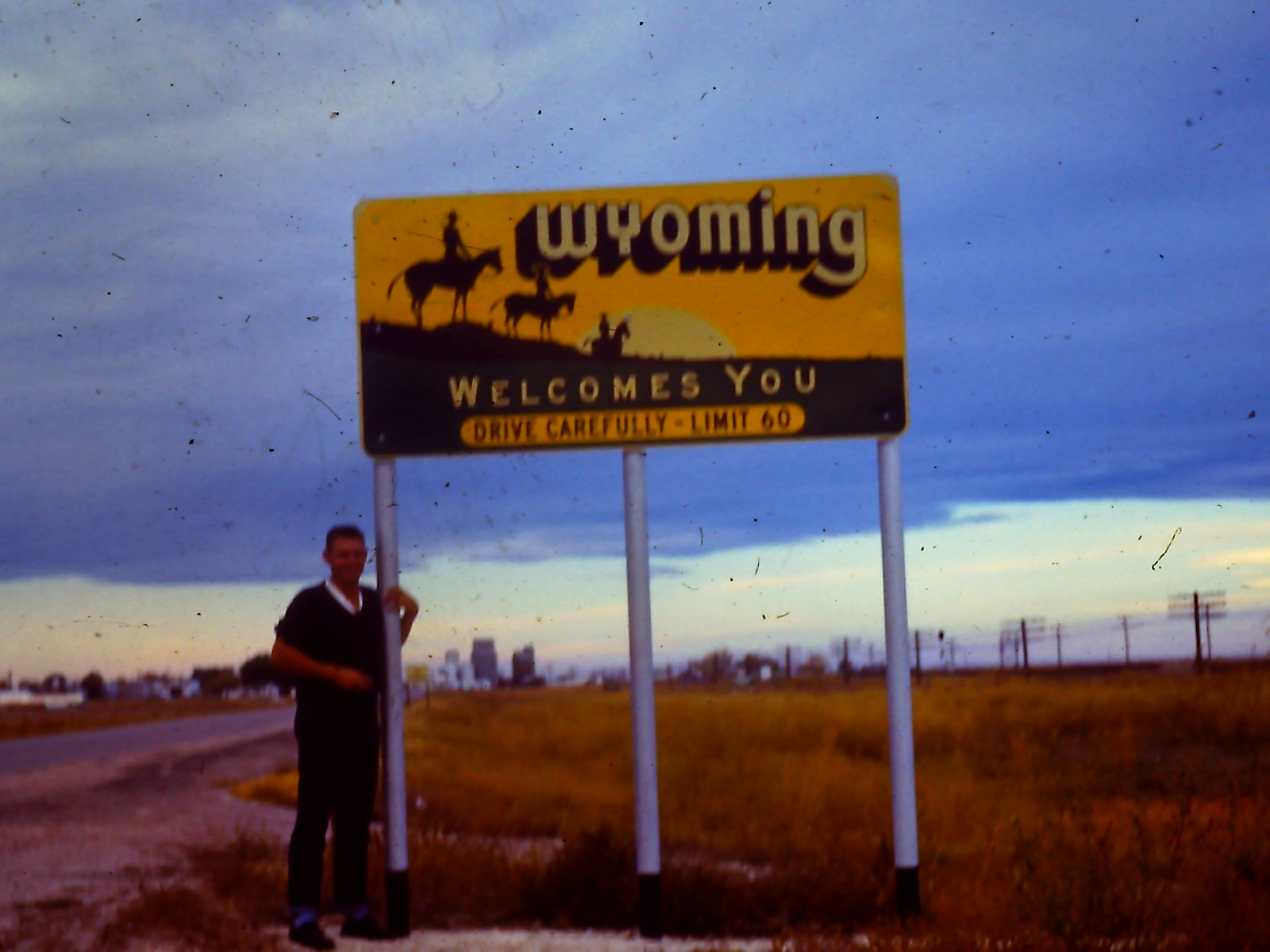This grainy, weathered photograph, possibly from the 1970s or 80s, captures a young man standing at the side of a rural road, gently grasping one of the three signposts supporting a large yellow sign. The sign, adorned with the silhouettes of three horsemen against a sunset backdrop, warmly announces, "Wyoming welcomes you." Beneath this greeting, in smaller text, it advises, "Drive carefully," with a speed limit of 60. The man, wearing dark clothing accented by a white collared shirt, stands amidst a landscape of expansive dark brown shrubs and a distant fence line. The sky above is a mix of blue and whitish hues, transitioning to darker, more ominous clouds. In the far background, tall buildings possibly hint at a distant cityscape, adding depth to the rural scene. The image, marred with small scratches and signs of age, evokes a sense of timelessness and nostalgia.